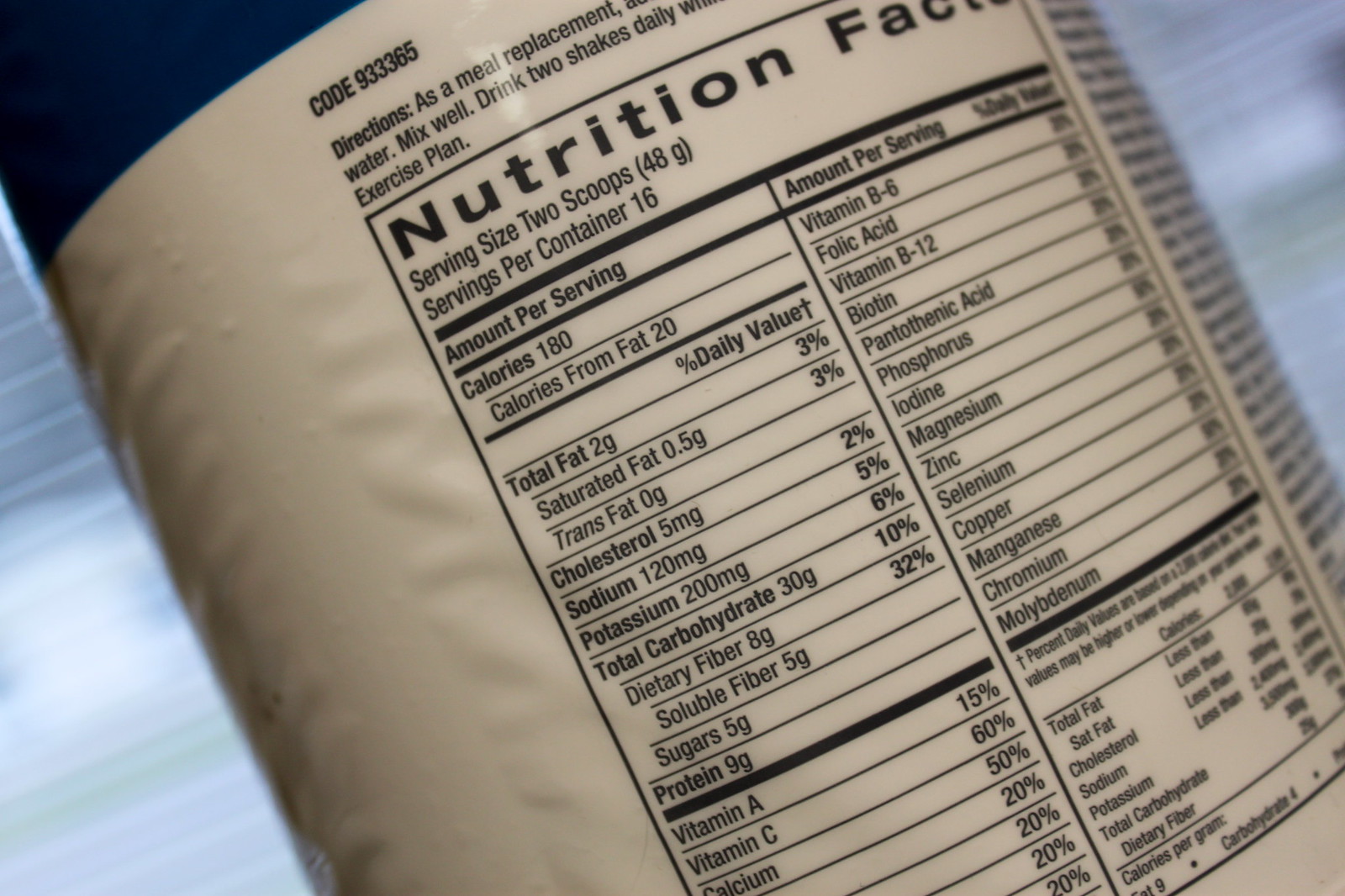The image prominently features a close-up shot of the nutritional information label on a dark brown jar or bottle of meal replacement powder. The label, which is angled at approximately 30 degrees off the vertical, is white and clearly states "Nutrition Facts" at the top. The serving size is noted as two scoops, with 16 servings per container. It provides detailed nutritional information, including 180 calories per serving, with 20 calories from fat, 2 grams of total fat, 5 milligrams of cholesterol, 120 milligrams of sodium, 200 milligrams of potassium, 300 grams of total carbohydrates, 8 grams of dietary fiber (including 5 grams of soluble fiber), 5 grams of sugar, and 9 grams of protein. Additional vitamins and minerals are also listed on the right-hand side of the label.

The background reveals window blinds, which are down but allow some light to filter through, hinting at an outdoor scene with a strip of green grass and possibly a house across the street. The image appears to be taken indoors, with the bottle placed in front of a window, providing a slightly blurry backdrop. The text on the label also includes usage instructions, mentioning that the product should be mixed with water, consumed as two shakes daily, and accompanied by an exercise plan. The close-up nature of the photograph ensures that the nutritional details are the primary focus, with other elements of the scene largely out of focus.